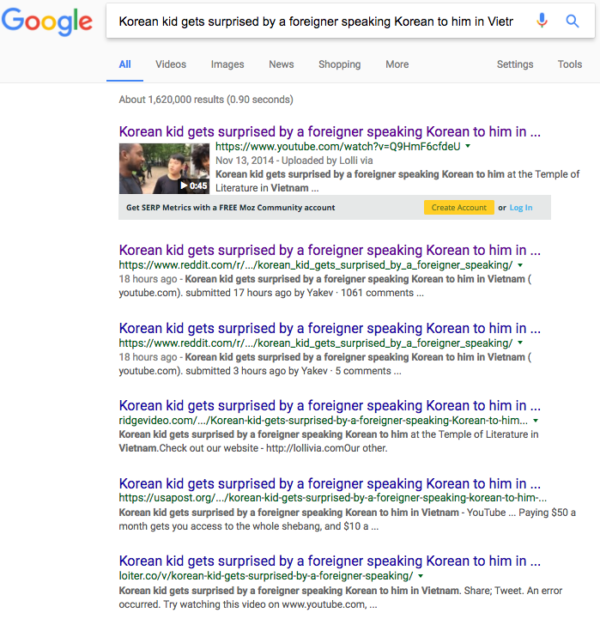The image displays a Google search results page. In the upper left, the iconic "Google" logo is prominently featured in its traditional colors of blue, red, yellow, and green. Below the logo, there is a large search bar containing the search query "Korean kid gets surprised by a foreigner speaking Korean to him." The search results reveal approximately 1,620,000 entries found in just 0.90 seconds.

The first clickable link matches the search query precisely: "Korean kid gets surprised by a foreigner speaking Korean to him." This specific link directs to a 45-second video hosted on YouTube, showing two men engaged in conversation. 

Below the initial link, the same headline appears five more times across various websites, including twice on Reddit, once on Ridge Video, once on USA Post, and once on LOITER.co. Each of these links directs to the same video, reiterating the widespread availability and popularity of the clip. Additionally, there are options to create an account or log in to access more features or engage with the content.